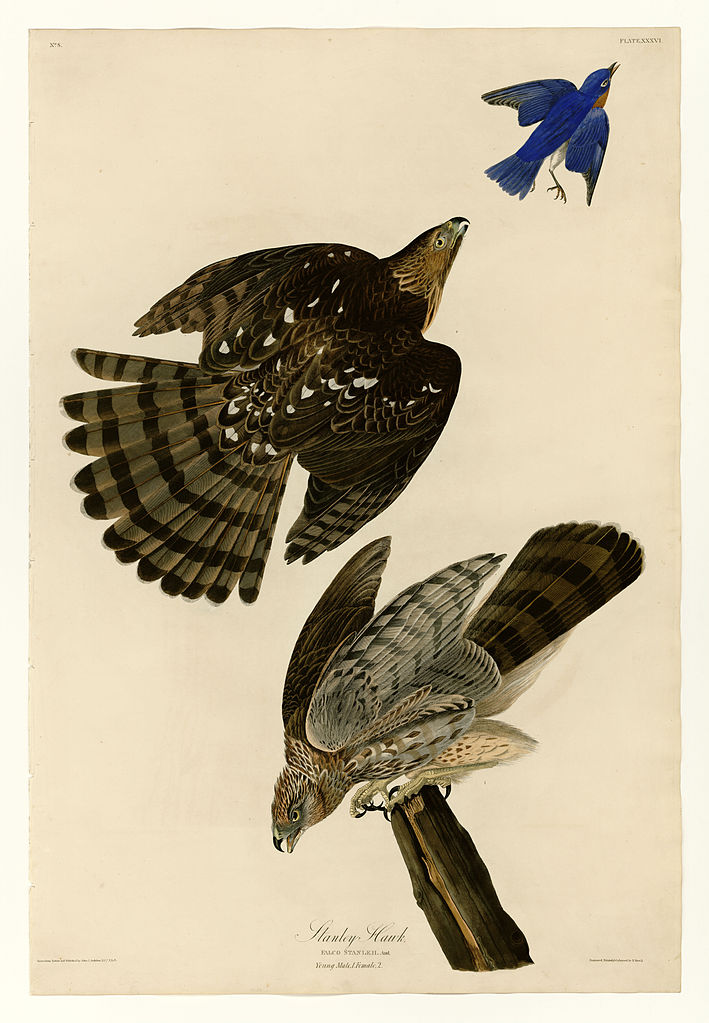The image is an intricately detailed drawing of three birds, reminiscent of illustrations found in classic natural science books. In the upper right corner, a small blue bird with striking yellow eyes is depicted in flight, seemingly fleeing from a larger bird of prey. This raptor, likely a hawk, has its wings partially drawn in, suggesting mid-dive motion despite appearing to ascend. It boasts predominantly brown feathers with dark lines and some white spots, creating a pattern on its shoulders and wings. Below this action scene, another raptor perches on a branch, looking downward with a partially open beak, adding a sense of intensity. This bird displays a palette of gray, black, brown, and yellow on the underside, and its tail is mostly concealed. The entire scene is set against a plain, off-white background, with a small, almost unreadable script in the bottom middle, enhancing its vintage scientific illustration aesthetic.